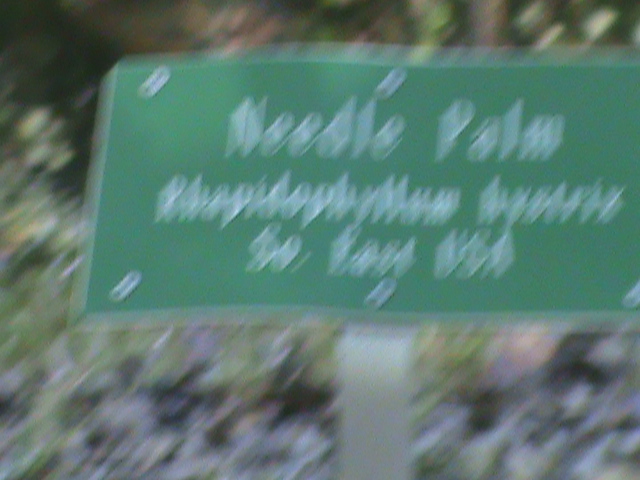This photograph depicts an extremely blurry green road sign attached to a whitish-brown wooden post or beam. The sign appears rectangular and bears the text "needle palm" in a thin, white sans-serif font, though the rest of the text is indiscernible due to the blurriness. At each of the top corners and in the middle of the sign, there are small white tabs. The background of the image features various types of vegetation, including trees, foliage, bushes, and possibly flowers in shades of green, purple, and white, though the details are unclear due to the overall blur suggesting possible camera movement when the picture was taken.